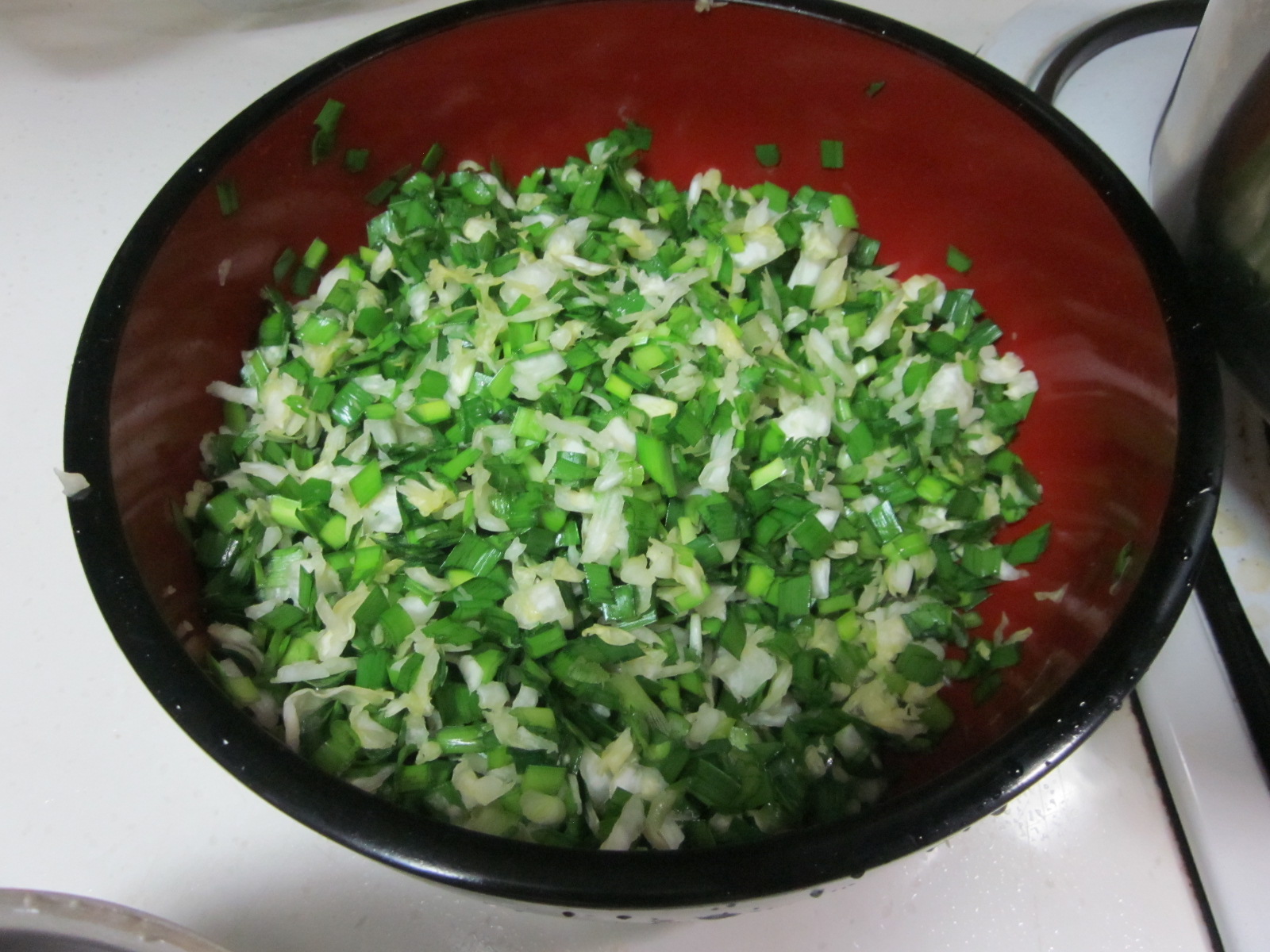The image captures a close-up of a glossy, rich blood-red bowl with a black trim rim, filled with finely chopped vegetables. The bowl is situated on a white countertop, adjacent to a stove with a silver pan on it, and a gray plate visible in one corner. Inside the bowl, there is a colorful mix of vegetables including white onions, green onions, edamame, and possibly some leafy herbs. The vegetables appear fresh, glistening with moisture or oil, suggesting they are prepped and ready to be added to a stir-fry dish. The bowl itself is somewhat see-through but maintains a dark shade of red. In the background, you can also see part of a white kitchen sink to the right, further situating the scene in a kitchen environment where cooking is in progress.